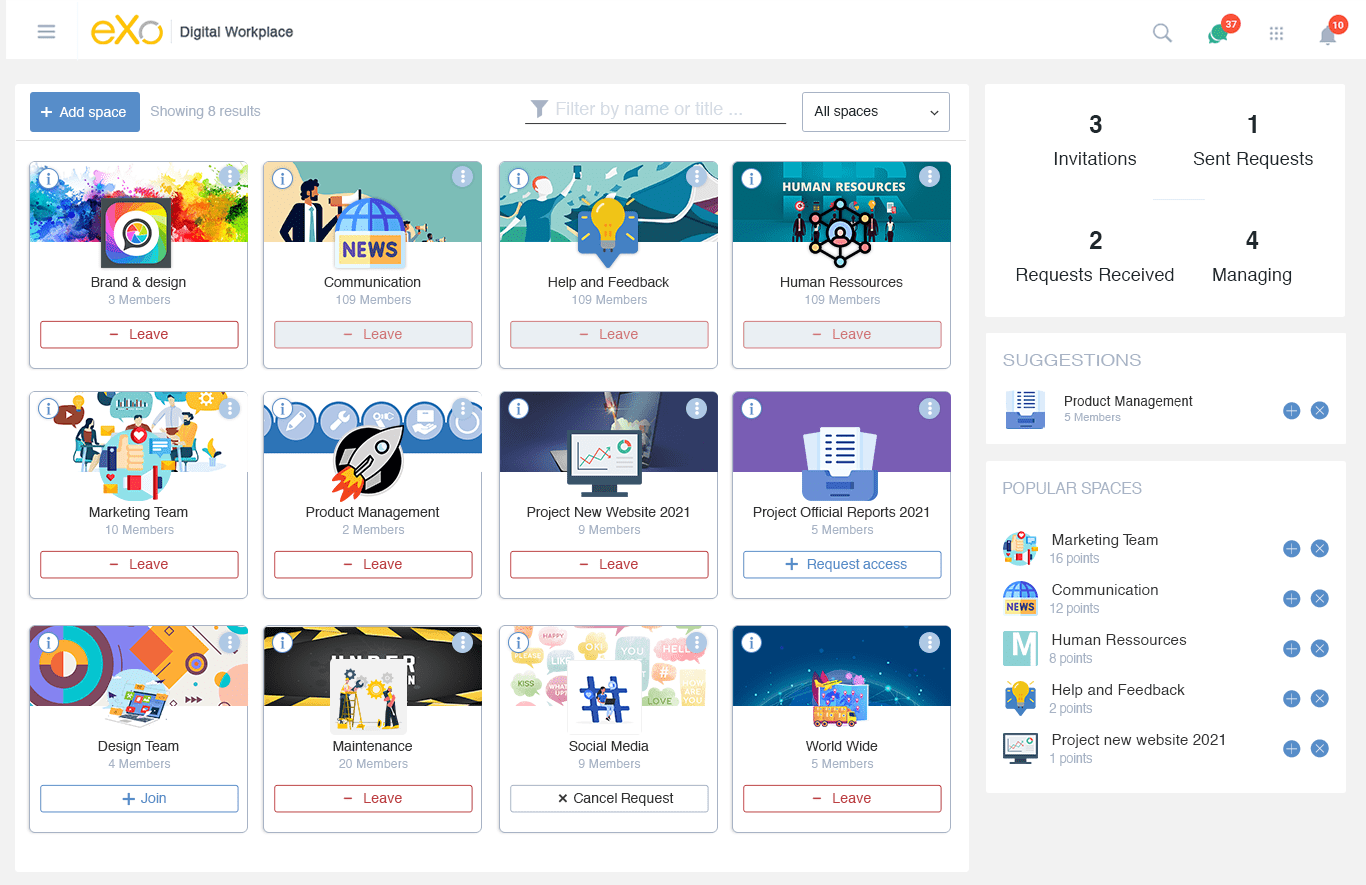The image depicts the homepage of the Dexile Digital Workplace, a platform hosted by the company EXO (spelled with a lowercase 'e', uppercase 'X', and a gold and gray 'O'). The EXO logo is situated in the top left corner next to a three-line hamburger menu icon. The website's primary font color is gold, with the 'O' in the logo being half gold and half gray, accompanied by the text "Digital Workplaces" to its right.

On the right-hand side of the header, there are several icons, including those for messaging and alerts, both marked with red circles displaying notification numbers. 

The main body of the page features a prominent blue button labeled "Add Space," characterized by a blue rectangle with a plus sign. Directly below it is a filter option labeled "Filter by name," positioned near the center. Adjacent to this is an "All Spaces" button with a drop-down menu.

The majority of the screen is occupied by a grid of 12 images, blending cartoonish computer clip art with specific titles and member information. Each tile follows a consistent format: the clip art at the top, a title such as "Brand Design," and a faded caption below indicating the number of members (e.g., "Three Members"). Each entry also includes a "Leave" button at the bottom.

On the far right side of the page, there is a box featuring sections for "Invitation Request," "Receive Request," and "Managing." Beneath this box, there are additional sections titled "Suggestions" and "Popular Spaces," each offering more selections and options for the user.